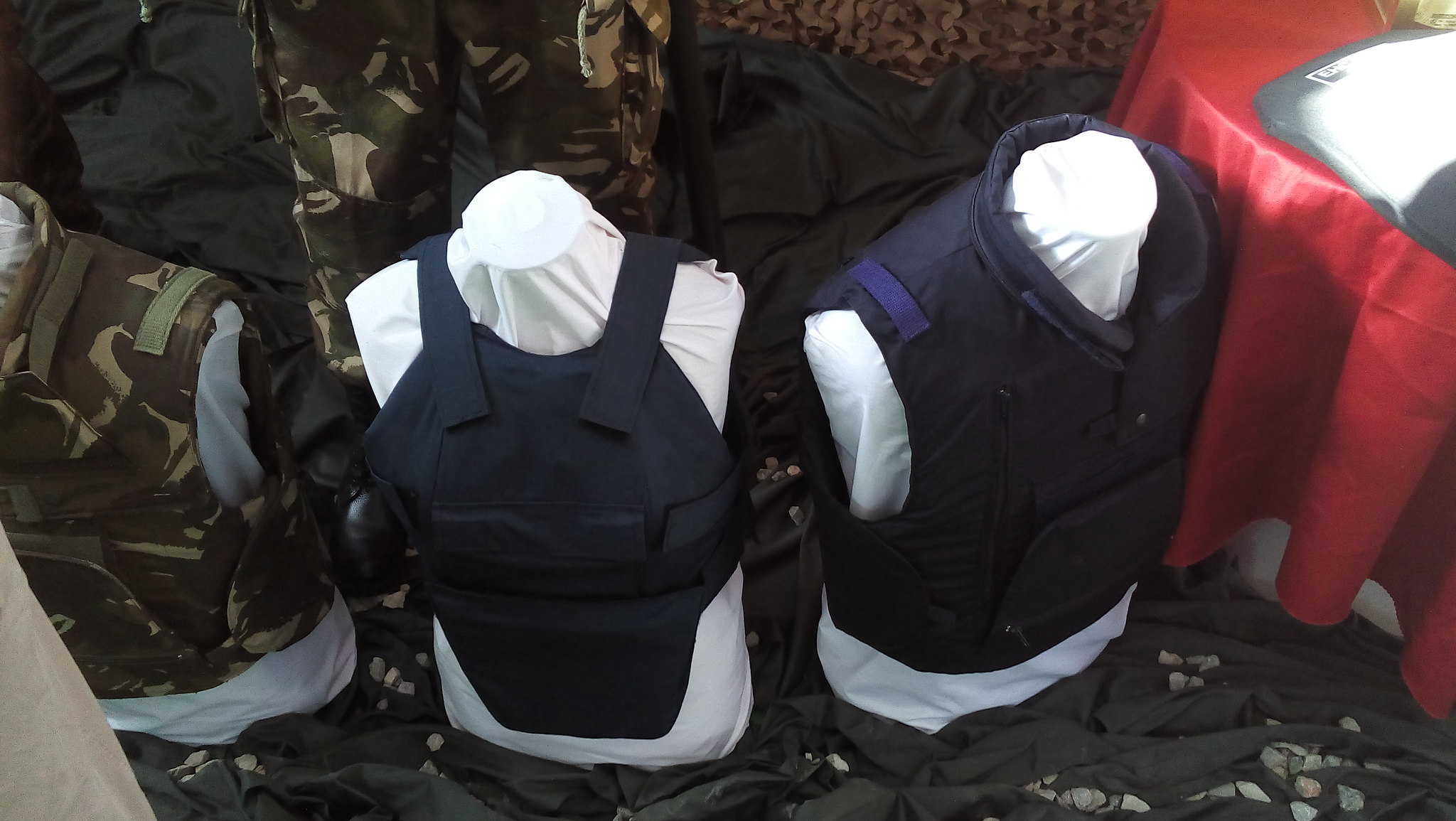In this photograph, three mannequins are displayed wearing various types of bulletproof vests. The leftmost mannequin is fitted with a brown-green-olive camouflage vest, offering full coverage around the torso. The mannequin in the center sports a distinctive black vest that leaves the flanks and much of the shoulders exposed, featuring lighter straps around the neck and minimal stomach protection. The third mannequin on the right is clad in a more substantial black vest, which covers the shoulders and includes a dark blue strap near the collar area.

All three mannequins are partially covered with white cloth torsos. In the background, a mix of clothing items can be seen, including a pair of camouflage-patterned pants matching the leftmost vest laid out on the ground. Additionally, to the right side of the photo, there is a table draped with a red tablecloth, beneath which some gray fabric is visible. Sunlight is also filtering through the right side of the frame, casting light on the setup but leaving the specific details somewhat obscured. The overall scene appears to be in a store or display setting focusing on body armor.